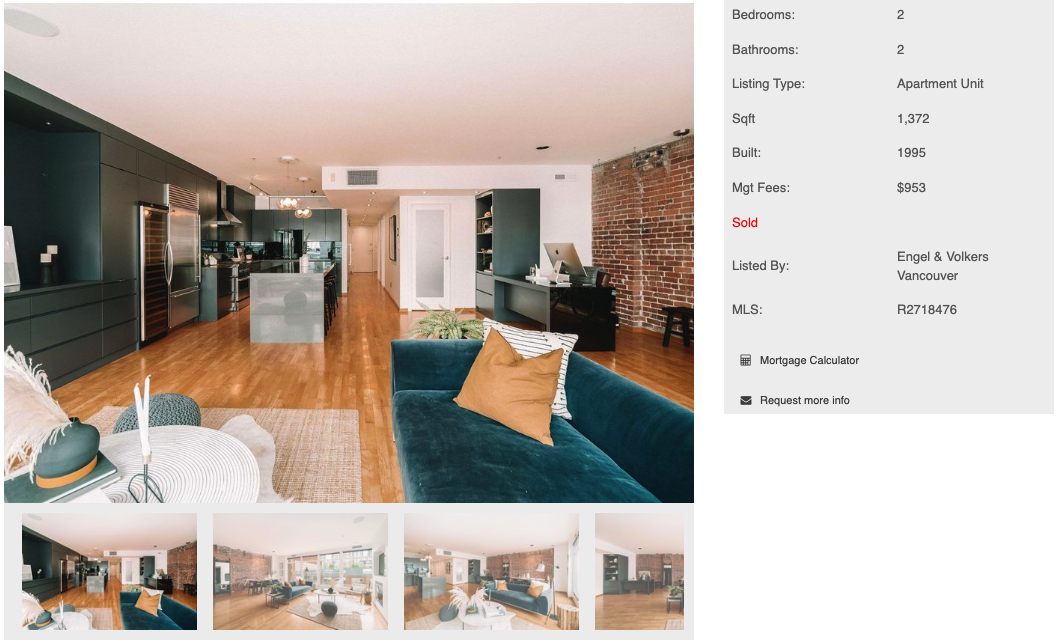This image is a detailed screenshot of a real estate web page showcasing the interior of a modern loft apartment. The living space features a white ceiling and a striking red brick wall on the right. In the foreground, there is a cozy living room with a blue velvet couch adorned with an orange-brown throw pillow and a white throw pillow with stripes. On the wooden floor, a circular coffee table is centered, decorated with candlesticks, books, and a hat. A mesh-like rug lies beneath the table.

The open-concept design flows into a modern kitchen on the left, equipped with sleek black cabinetry and a stylish kitchen island with chairs neatly placed underneath. A silver refrigerator stands prominently in the kitchen, while hanging lights illuminate the space.

Towards the back, a black stool and a black desk with an Apple desktop computer are positioned against the red brick wall, with a black bookshelf visible behind them. A bit of the hallway leads further into the apartment. The kitchen's modern design is complemented by a contemporary living area, blending functionality with style.

On the right-hand side of the image, a gray information box provides additional details about the property: 
- Bedrooms: 2
- Bathrooms: 2
- Listing Type: Apartment Unit
- Square Feet: 1,372
- Built: 1995
- Management Fees: $953
- Sold listed by: Engel & Völkers Vancouver
- MLS: R2718476